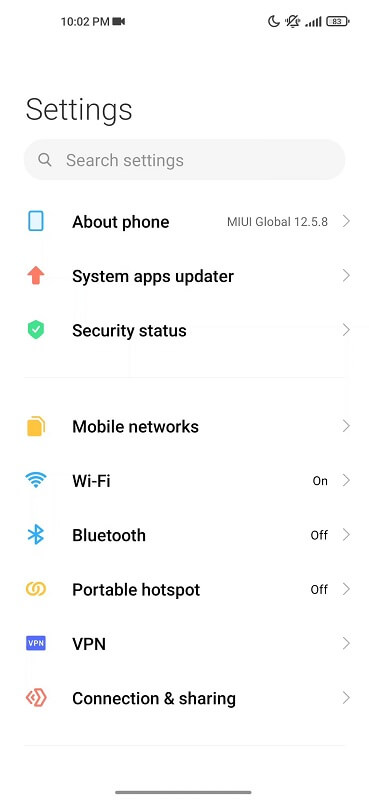The image captures a detailed view of a cell phone screen displaying the settings menu at 10:02 p.m. The top-left corner shows the current time and a video camera icon. Meanwhile, the top-right corner displays a moon icon, indicating a "Do Not Disturb" status, a bell icon with a line through it, a cellular connection signal, and a battery icon with "83%" remaining charge.

Directly beneath, the screen header reads "Settings" in large print. A search box featuring a magnifying glass icon and the text "Search settings" resides just below. Further down, on the left, an icon of a phone accompanied by the text "About phone" and "MIUI Global 12.5.8" is visible. Adjacent to this is a red upward-pointing arrow labeled "System apps updater."

Proceeding further, a badge with a green background and a white checkmark centers the text "Security status." Below, a yellow square icon is labeled "Mobile networks," followed by a blue wireless signal icon next to "Wi-Fi," which indicates "On" to its right. Continuing downward, a blue Bluetooth logo appears beside "Bluetooth," with a status of "Off." Two interlocking rings signify the "Portable hotspot," also marked "Off."

The subsequent section features a rectangle with the letters "VPN" next to the text "VPN" and terminates with a red icon labeled "Connection and sharing."